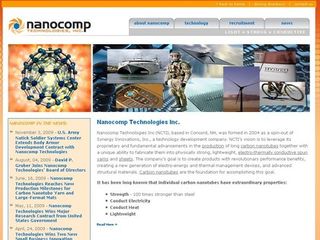A screenshot of a company webpage features prominently in the upper left corner, the distinctive Nanocomp logo and brand name. Despite efforts to enlarge the image, the text remains largely unreadable due to blurriness, making the finer details of the company’s mission or services unclear. Visible below the logo is the title "Nanocomp Technologies, Inc.," yet the accompanying description is equally indecipherable. The left side of the image showcases an illustration resembling an atom set against a red, white, and orange tie-dye backdrop. On the right side, several images are arranged, including a large boat, a figure that could be a soldier or a robot (noticeably pixelated), an open cell phone, a wind turbine, and a bicycle. While the label beneath these pictures is legible and identifies the company as Nanocomp Technologies, Inc., the text providing further information remains too blurry to read, even after magnification. The background appears predominantly white, further emphasizing the text.